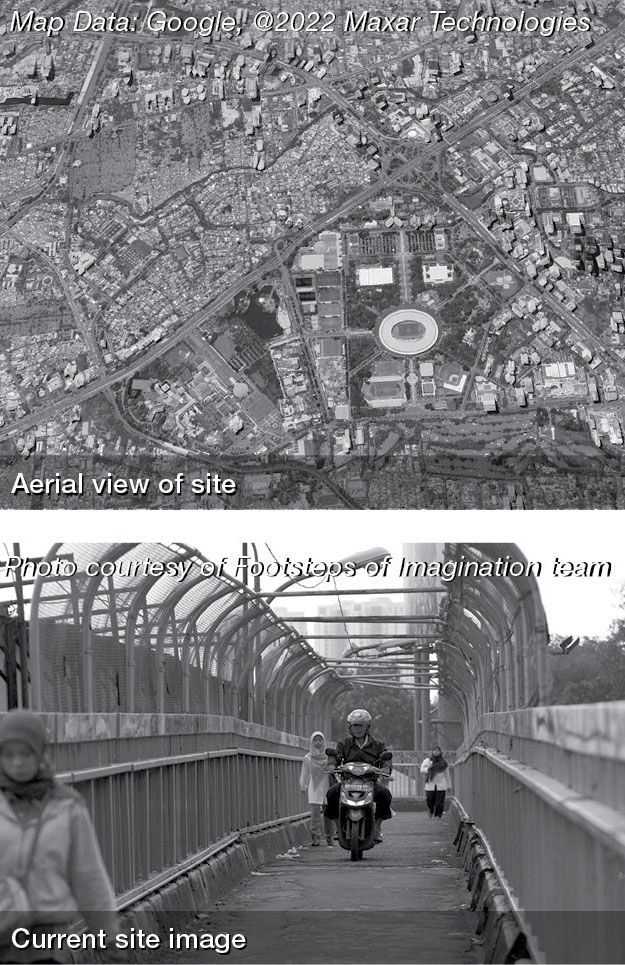The image contains two black-and-white panels, with an overarching theme of a site from both an aerial and ground perspective. The top panel presents an aerial view from Google Maps of what appears to be an urban or industrial area, complete with surrounding neighborhoods and a major roadway snaking through the layout. The large intersection near the center-right stands out, hinting at a significant infrastructure hub. The caption on this photo reads "Map Data, Google, 2022 Maxar Technologies," with an additional label at the bottom saying "Aerial View of Site."

Below, the bottom panel shifts to a ground-level perspective, capturing a scene of daily life. The scene shows a man riding a motorcycle or moped along an enclosed bridge, which is surrounded by fencing that arches halfway up the sides. Accompanying him are several pedestrians, specifically a woman in front and two women behind him, all adorned in traditional head coverings, suggesting cultural attire perhaps from the Far East or a Muslim region. The text on this photo credits the "Footsteps of Imagination Team" and labels the image as the "Current Site Image."